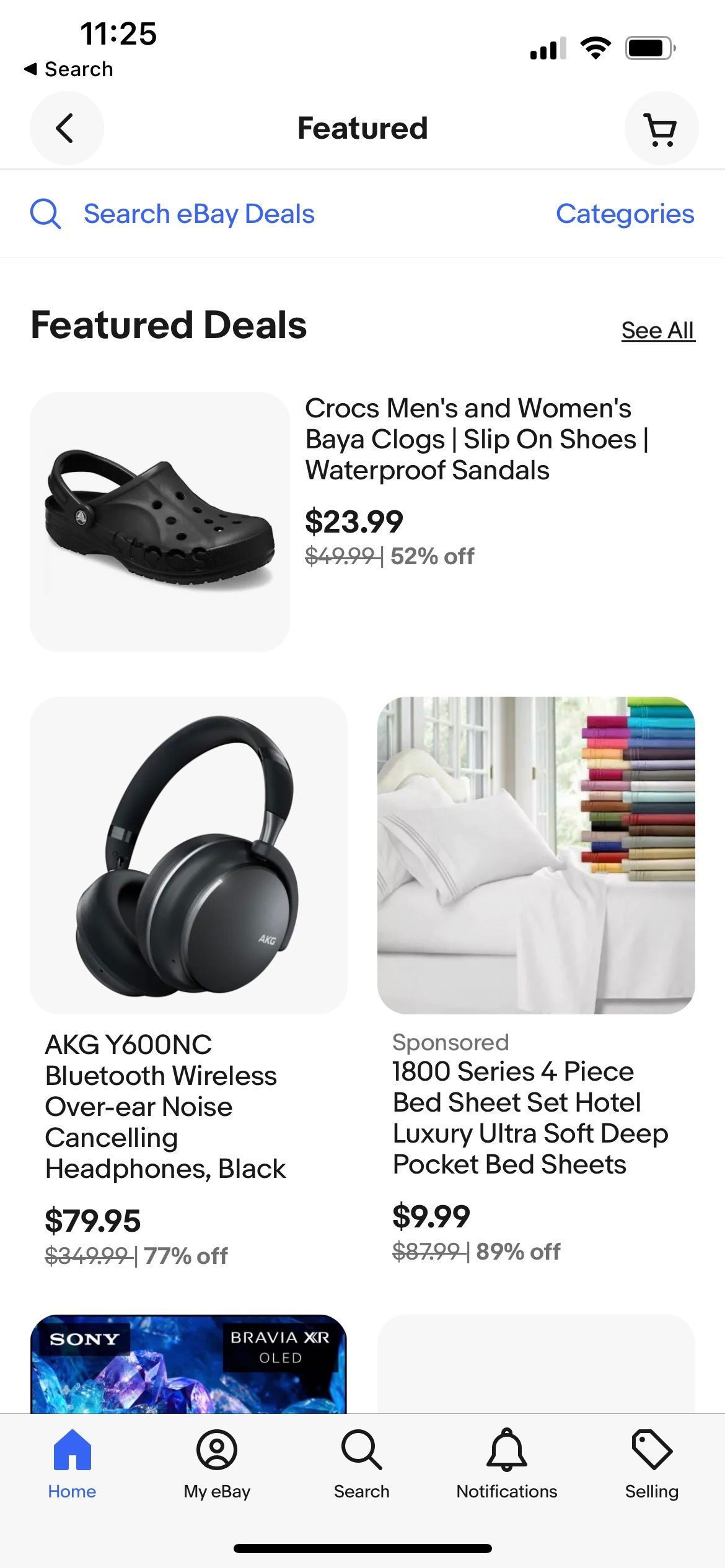The image appears to be a vertical screenshot taken from a smartphone displaying the eBay app interface against a white background. Detailed elements of the screen include:

**Upper Section:**
- Top left: The time is displayed as 11:25 in black text.
- Top right: Signal strength, Wi-Fi icon, and battery life indicator are visible.

**Header:** 
- Below the time, there is a "search" bar with a small arrow next to "featured" in bold, centered. 
- On the right is a shopping cart icon. 
- A thin gray line separates this section. Below it, a blue magnifying glass icon appears with the text "Search eBay deals." To the right, "categories" in blue text.

**Main Content:**
- Under *Featured Deals* (bold text):
  - **Crocs Men's and Women's Clog Slip-On Shoes**: Waterproof sandals priced at $23.99, marked as 52% off.
  - A link that says "see all."
  - **Bluetooth Wireless Over-Ear Noise-Cancelling Headphones**: In black, originally $79.95, now 77% off.
  - **1800 Series Four-Piece Bedsheets**: Hotel luxury ultra-soft deep pocket bedsheets priced at $9.99, discounted by 89%.

**Cut-off Ad:** 
 A partially visible advertisement for a Sony product at the bottom of the listing section.

**Footer:**
- eBay navigation buttons: "Home" (highlighted in blue), "My eBay", "Search", "Notifications", and "Selling".

Each section and item is distinctly separated, providing a clear and structured layout of the eBay app’s featured deals.